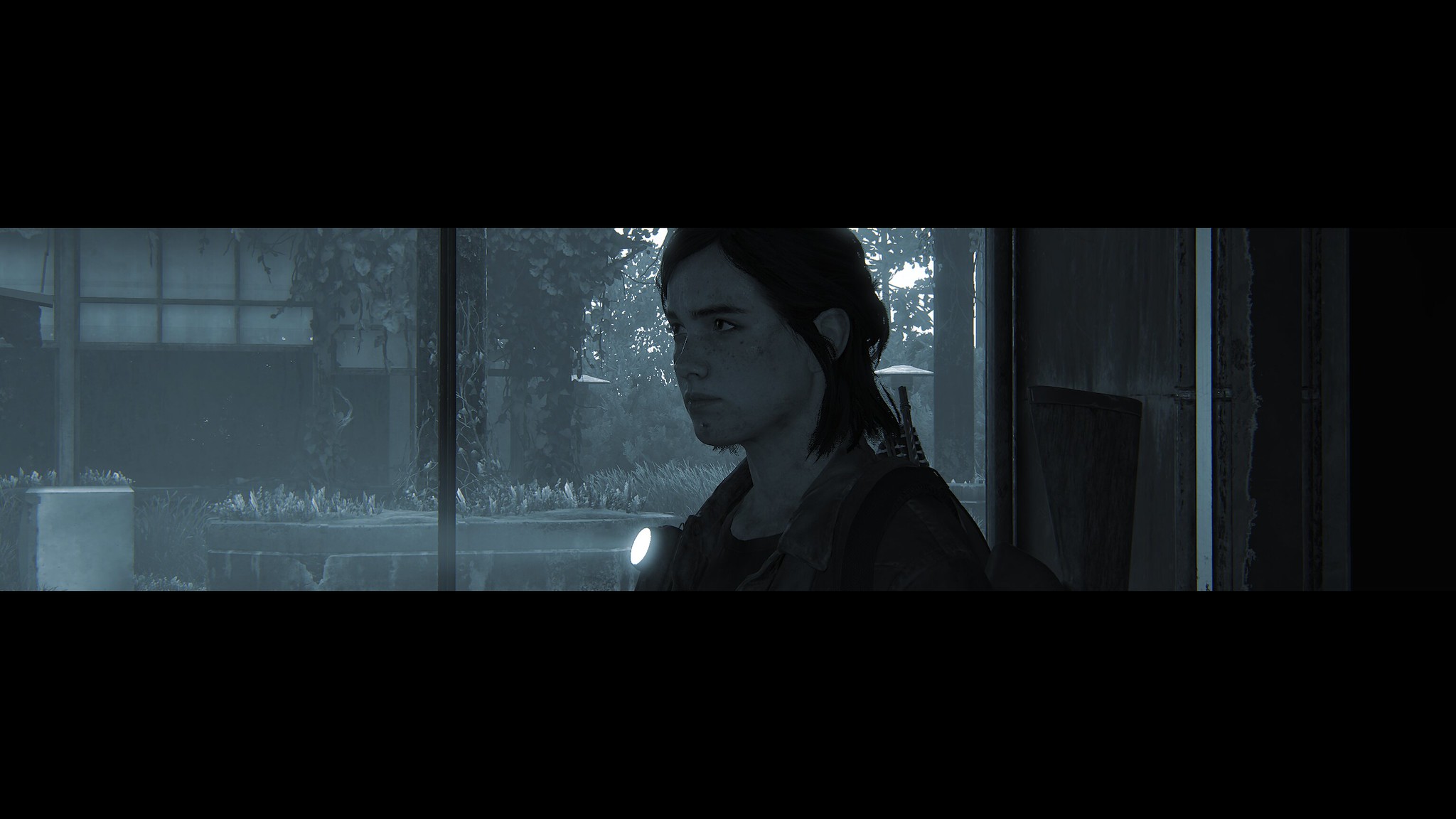The image is a landscape-format screenshot from a video game, likely "The Last of Us," presenting a highly atmospheric and eerie scene. The image is framed by two large black bars at the top and bottom, making up approximately half of the entire picture area. In the center, a woman with short dark hair and a dark complexion, accentuated by dim lighting, sits in front of two large window panes. She is not looking out of the window, but rather parallel to it, towards the left side of the frame. She is wearing a brownish jacket over a dark shirt, and there is a flashlight attached to her right side, possibly near her backpack strap or held in her hand. The windows reveal a dark and possibly rainy outdoor scene, where foliage and trees dominate, with ivy—or similar vines—hanging prominently. A building can be faintly seen across the way, adding to the overgrown, post-apocalyptic atmosphere of the setting.